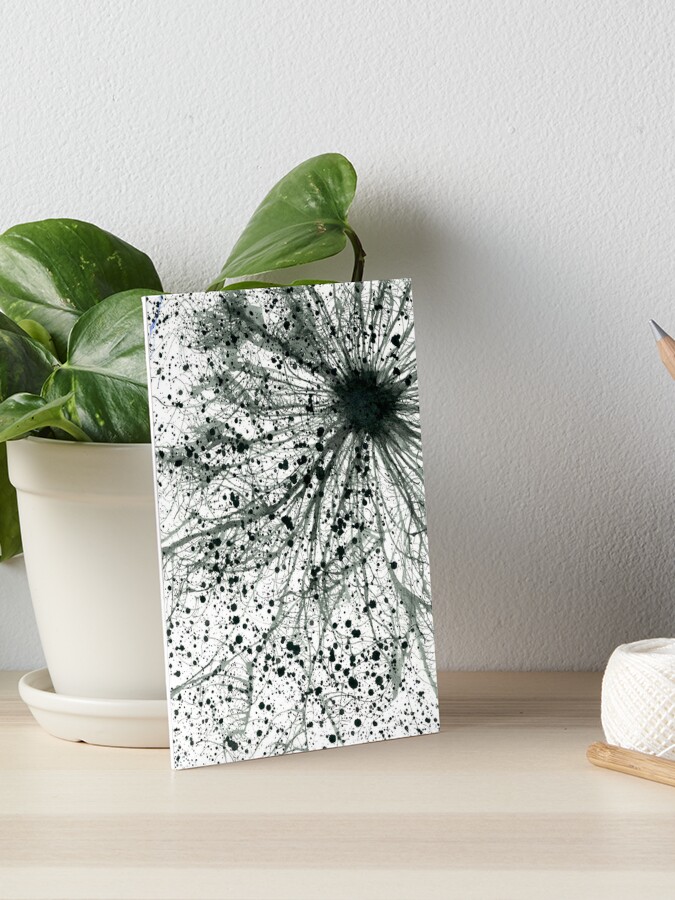The photograph captures a detailed interior scene featuring a large houseplant with broad, heart-shaped green leaves, potted in an off-white ceramic planter that sits on a small white tray. The floor is covered in white gravel, bordered by a tan molding where the wall meets the floor. Five feet to the right of the plant, a small, abstract black-and-white painting leans against the planter. The painting, on a rectangular canvas with vertical sides twice as long as the horizontal, depicts a large black dot near the top-right corner, from which numerous black lines emanate in all directions, resembling a burst or a brain synapse. The white background of the painting is splattered with speckles of black paint, creating a dynamic, energetic effect. The wall behind casts dark gray shadows that add depth to the scene.